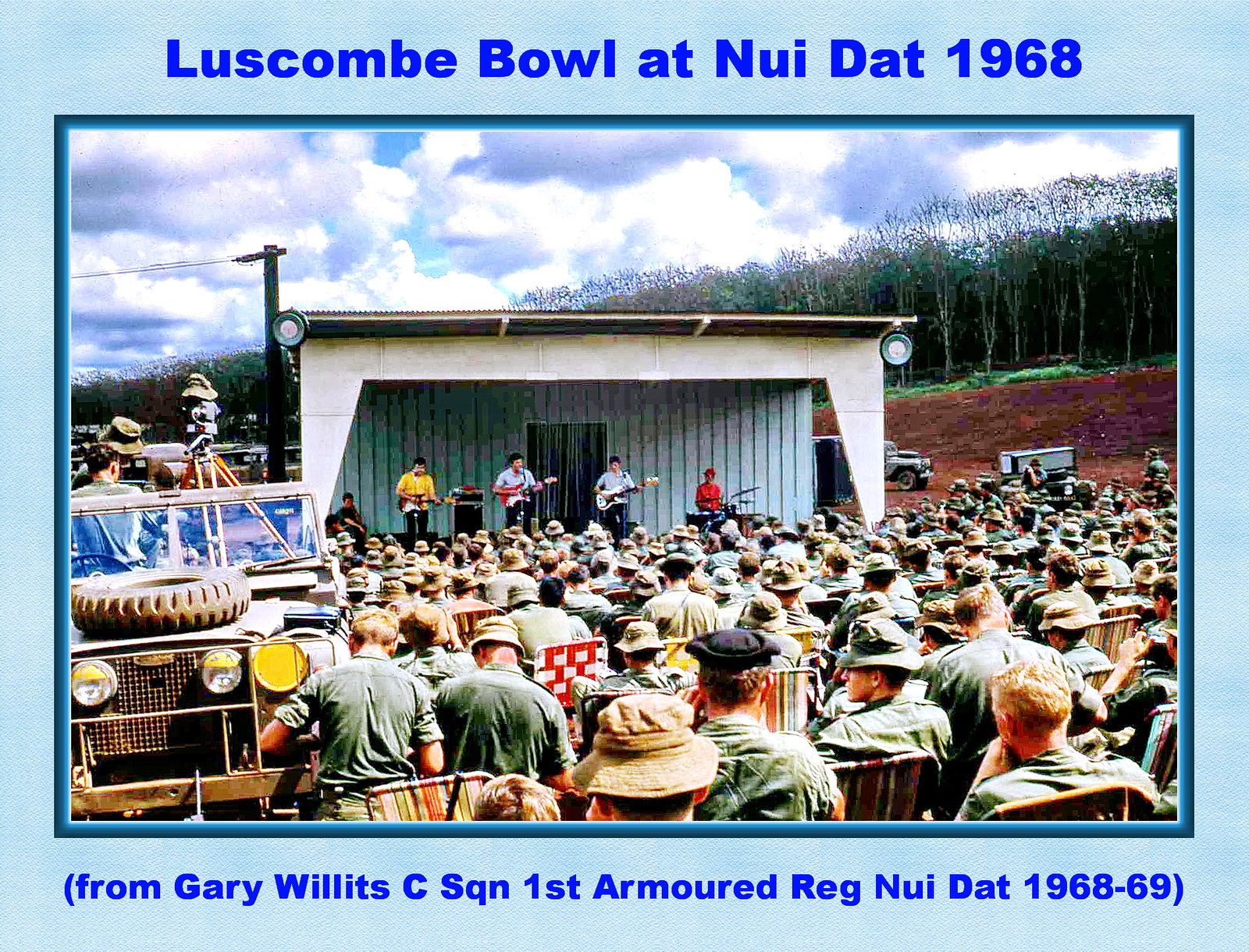The photograph captures a distant shot of a concert held during the Vietnam War at Luscombe Bowl, Nui Dat, in 1968. The stage, set up with a canopy and flanked by speakers on the top right and left, features several performers with guitars and a drummer situated towards the right, identifiable by their red shirt and red hat. The stage, more like the porch of a building, is backed by a blue background and the surrounding field extends into thick woods with tall trees. In front of the stage, a large audience of soldiers, dressed predominantly in green shirts and khaki military garb, is seated on field chairs. To the far left of the audience, a military Jeep is visible. The scene unfolds under a cloudy yet bright sky. Above the photograph, dark blue lettering reads "Luscombe Bowl at Nui Dat 1968," while at the bottom, in similar dark blue lettering, appears the credit: "From Gary Willits, C Squadron, 1st Armored Regiment, Nui Dat 1968-69."